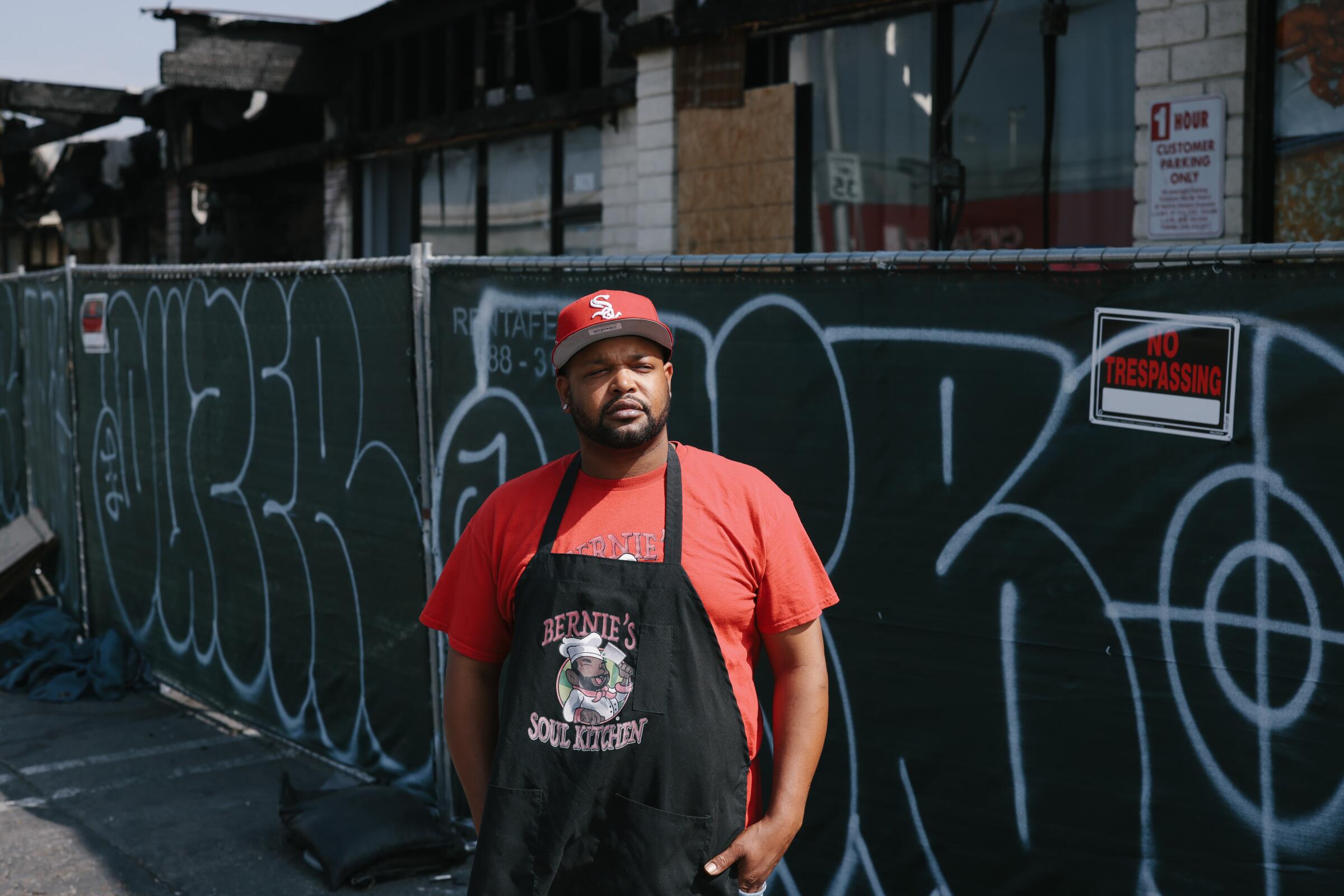The photograph depicts a determined-looking African-American man standing in front of a chain-link fence covered with green banners that have spray-painted graffiti and a "No Trespassing" sign. He is wearing a red baseball cap with a white "S" on the front, a matching red short-sleeved shirt, and a black apron emblazoned with the logo of Bernie's Soul Kitchen. The apron features a caricature of the man himself, dressed in a chef's outfit, complete with his distinctive beard and face shape. His hands are in his pockets, and he is squinting slightly against the sun's glare. Behind the fence, there are shops with some boarded-up windows, suggesting an area in need of revitalization.